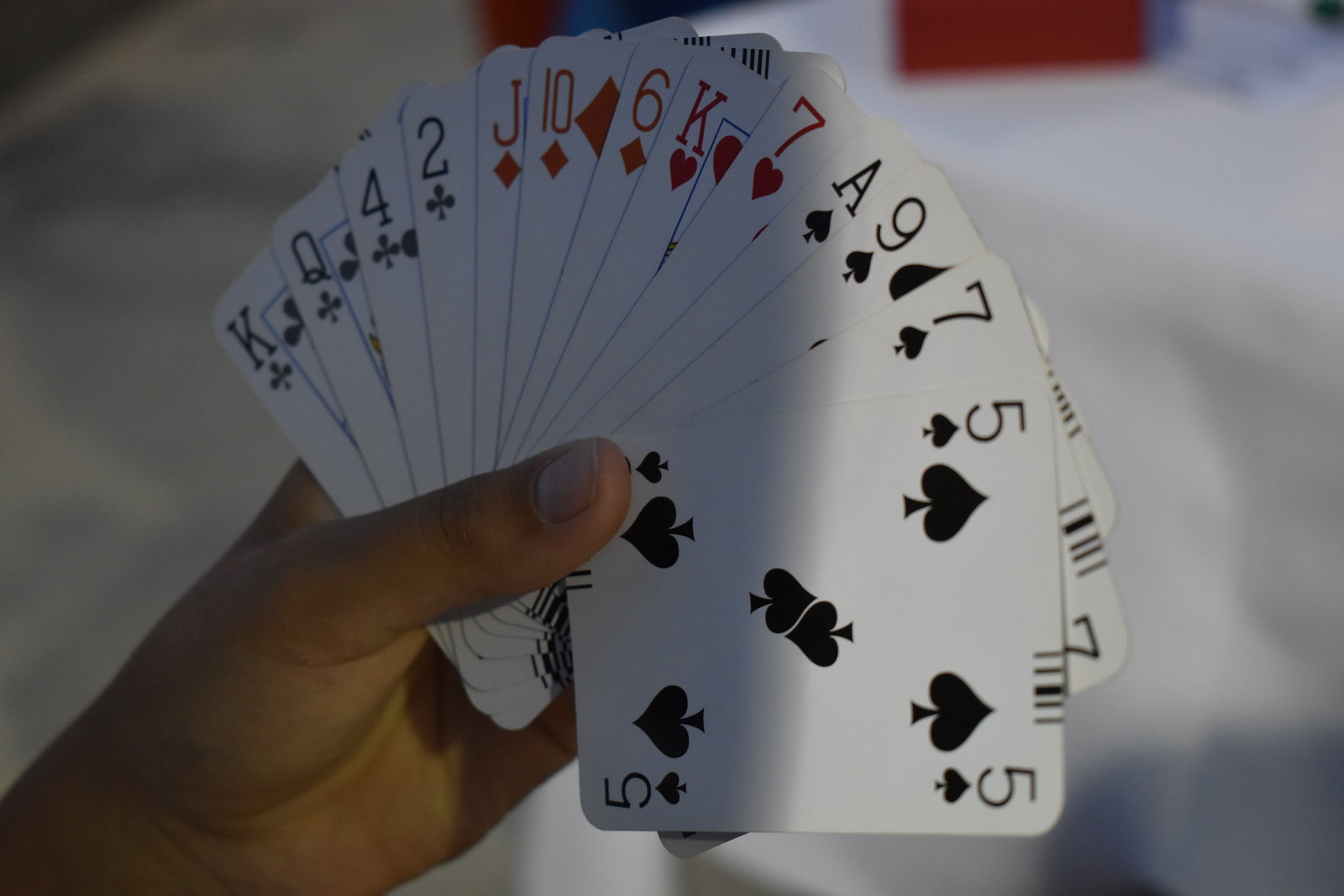In this slightly blurry image, the left side features a shadowy area with mingled shades of dark and light gray. A hand, prominently positioned in the foreground, clutches a substantial fan of playing cards. These cards, set against a white background, include a diverse array: King, Queen, Four, Two, Jack, Ten, Six, King again, Seven, Ace, Nine, another Seven, and Five. Each card displays its rank and suit, while the face cards are adorned with intricate blue lines framing the regal depictions of Kings, Queens, and Jacks. The scene is set on a white table, at the end of which rests a small wooden box. On the right side, sunlight streams in, casting a gentle glow on the top edges of the cards, enhancing their crisp, white backgrounds.